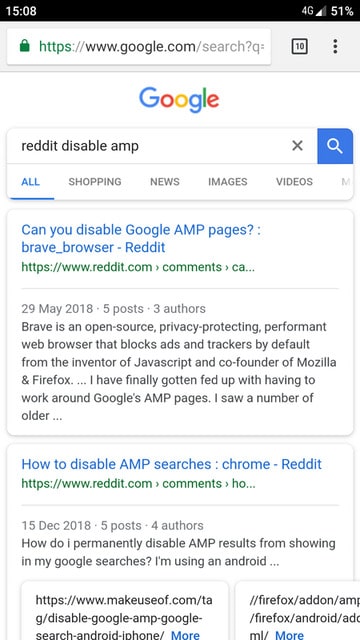This image is a detailed screenshot from a smartphone, showcasing a Google search results page. The top border of the screen is black and features key status indicators. On the left side, the time is displayed in white as 15:08. On the right side, icons indicate a 4G network connection, a wireless signal, and a battery level at 51%.

Beneath the status bar, the browser window is open to Google, with the URL partially visible as "google.com/search". Dominating the upper portion of the page is the Google logo, composed of a blue "G", red "O", yellow "O", blue lowercase "g", green "l", and red "e". Directly below the logo is the search box, containing the query "reddit disable amp".

The search results are displayed on a white background. The first result, highlighted in blue, has the headline: "Can you disable Google AMP pages Brave_Browser Reddit". Below this headline, separated by a light gray line, is additional information: dated 29 May 2018, it notes there are five posts on the topic. The description reads: "Brave is an open-source, privacy-protecting, performance-oriented web browser that blocks ads and trackers by default, from the inventor of JavaScript and co-founder of Mozilla and Firefox. I have finally gotten fed up with having to work around Google's AMP pages. I saw a number of older..."; the text is partially cut off.

The second search result, also in blue, reads: "How to disable AMP searches Chrome Reddit". Below it, dated 15 December 2018 with five posts and four authors, the snippet starts: "How do I permanently disable AMP results from showing in my Google searches? I'm using an Android..."; the rest of the text is not visible in the screenshot.